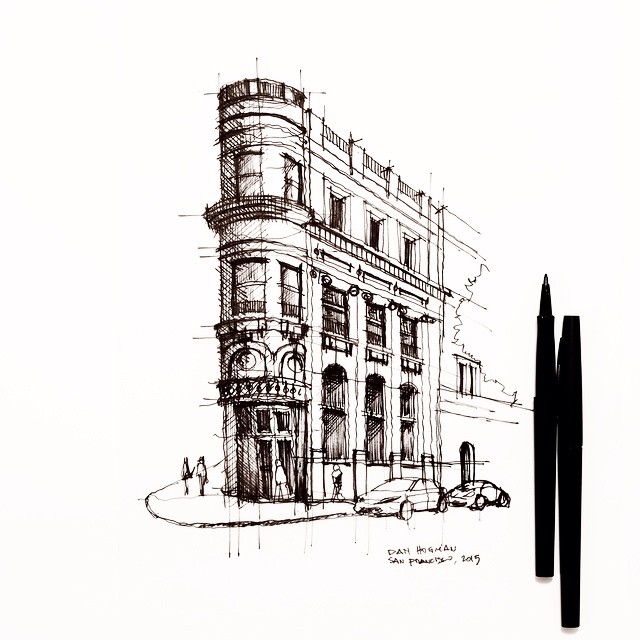This is a detailed line drawing of a three-story, triangular-shaped building reminiscent of the Flatiron Building in New York. The illustration is signed by Dan Hogman, labeled "San Francisco, 2015." The structure features ornate architecture with intricate filigrees and friezes. The building has a rounded turret on one end, elaborate arched windows on the ground floor, followed by two stories of standard windows above. At the top of the building is a flat roof with a railing, suggesting a rooftop deck. Two cars are parked beside the building, and a few small figures walk around it, adding a sense of scale. Notably, two women are depicted walking along the left side, and a man appears to be entering through a revolving door at the corner. The drawing also includes an adjacent, less detailed building. Additionally, to the right side of the image, there are two writing implements, possibly ink pens or mechanical pencils, on the white background. The overall style of the drawing is black and white, with varying levels of detail throughout.